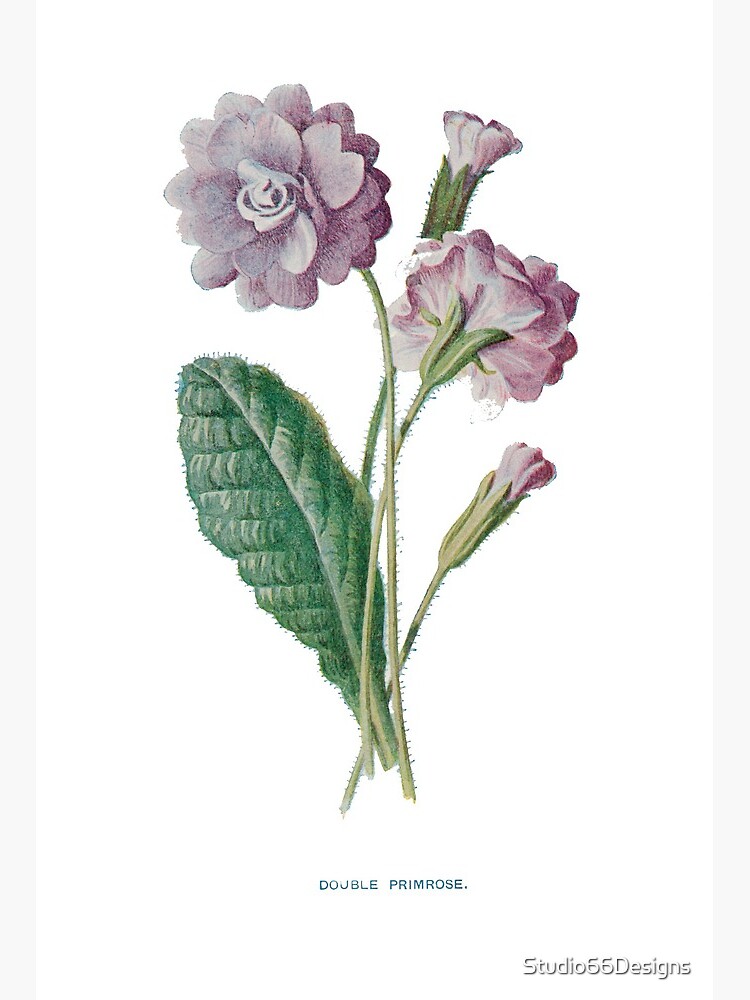This detailed color illustration of a double primrose, set against a white backdrop, captures the botanical beauty and intricacies of the flower. The artistic rendering features multiple views of the primrose—a fully bloomed flower facing the left, a partly visible rear view of another bloom, and several bud stages. The bloom is a striking blend of lilac with darker purple shades. The elongated green-gray stem is adorned with a single, medium-sized dark green leaf, characterized by its sharp ridges and tiny fuzzy parts extending onto the stem, likely a defense mechanism against predators. The buds, encased in green leaves with subtle purplish tips, are vividly depicted to show the progression from bud to full bloom. A watermark reading "Studio 66 Designs" is present at the bottom right, affirming the scientific and artistic merit of this botanical print.